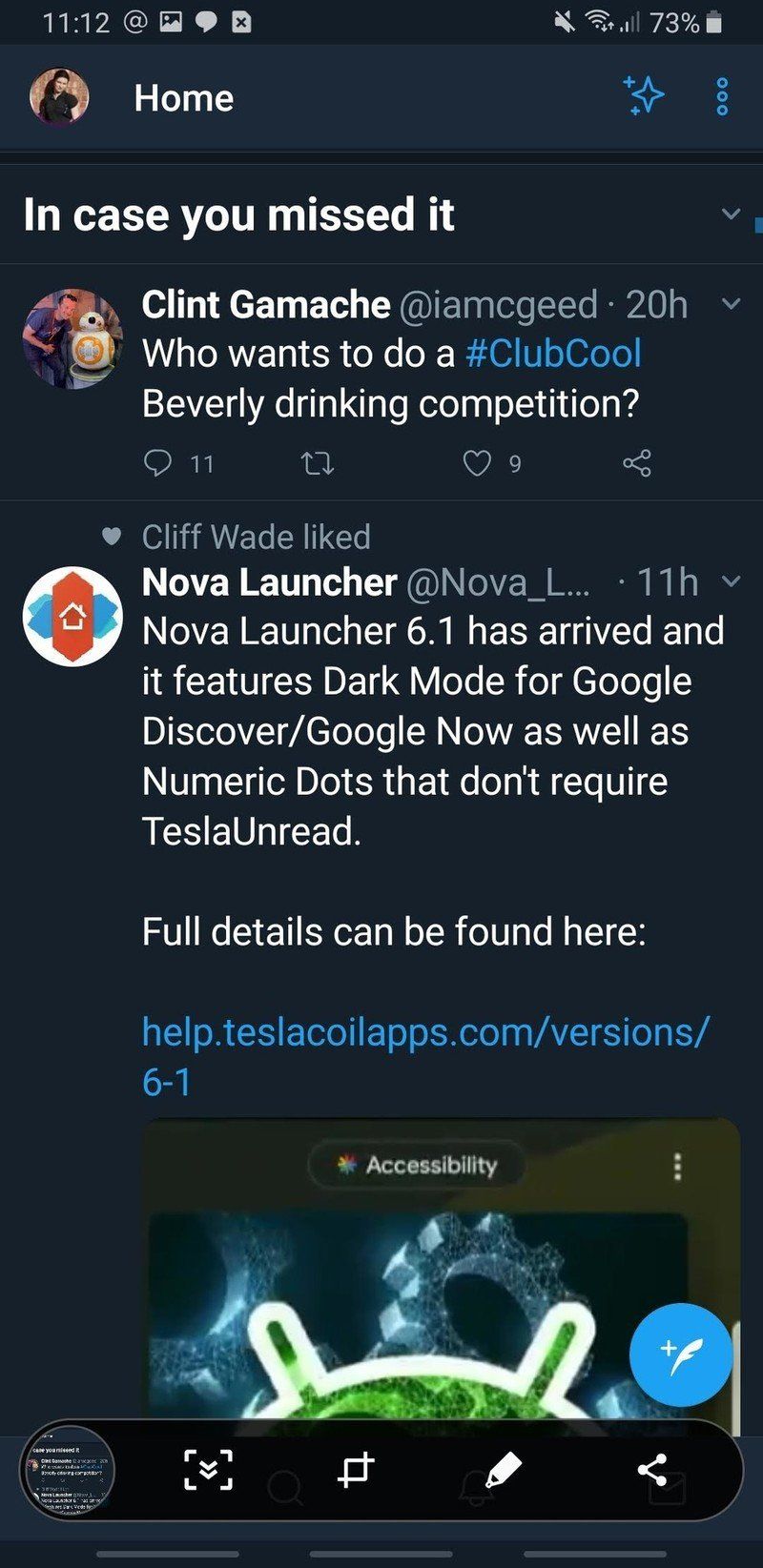A detailed caption for the image could be:

"This screenshot appears to be taken from a mobile device, specifically capturing the screen of a social media platform, most likely Twitter. At the very top of the screen, there is a status bar displaying the current date along with icons for various notifications and battery life. Directly below this, an interface section includes an avatar icon, a 'Home' button, and additional navigation icons.

The content starts with a section titled 'In case you missed it,' featuring recent posts. The first highlighted post is by a user named Clint Gamatch (@IMcGeeD) and was posted 20 hours ago. Clint's post reads, 'Who wants to do a #clubcool Beverly drinking competition?' This post has garnered 11 comments, 9 likes, but no reposts.

The subsequent post is from 'Nova Launcher' with the handle @Nova_L... and includes their avatar. The content announces the release of 'Nova Launcher 6.1,' highlighting new features such as dark mode for Google Discover and Google Now, as well as numeric dots that do not require Tesla Unread. Additional information is linked to their help site (help.teslacoilapps.com version 6.1).

Further down, the image of another post is partially visible but not clear enough to extract details. The bottom section of the screenshot displays standard image editing tools, including icons for editing, cropping, sharing, downloading, and a 'post' button, suggesting the user is on Twitter and has the option to create a new post.

Overall, the screenshot captures the interactive interface of a Twitter feed, showcasing various functionalities and user interactions within the social media platform."